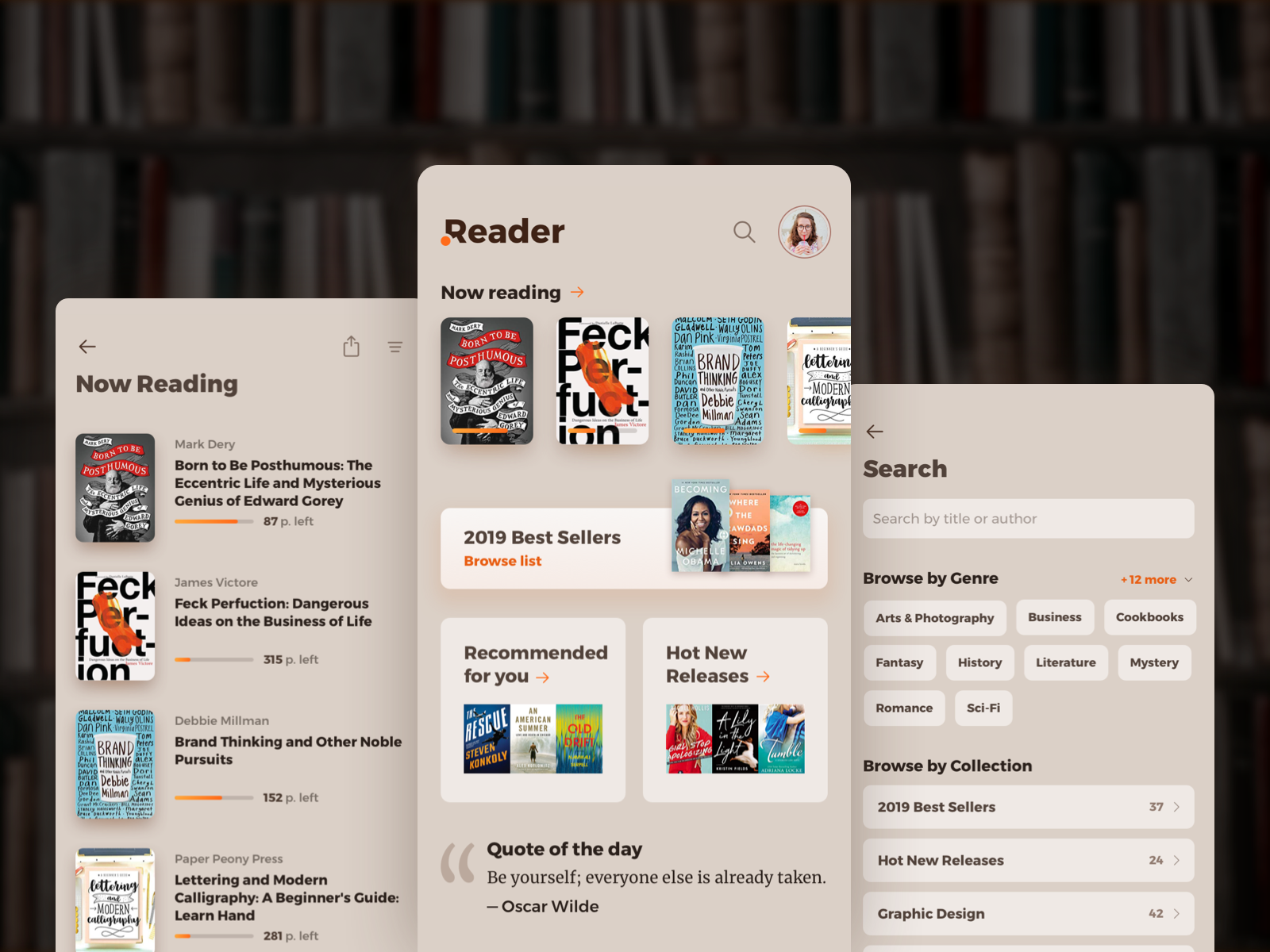This is an intricate image showcasing the interface of a book-reading application. The background is a softly blurred, black bookcase filled with books. The display consists of three overlapping screenshots from a smartphone utilizing the app. 

1. **Left Screenshot:**
   - **Top Section:** The background is tan. At the top left, "Now Reading" is prominently displayed in bold brown letters. The upper right corner contains an upload arrow and a button with three horizontal lines.
   - **Middle Section:** On the left, a gray icon features an older man flanked by red banners. The title "Born to be Posthumous: The Eccentric Life and Mysterious Genius of Edward Gorey" by Mark Dery is listed. Below it, there's a white book titled "Feck Perfection: Dangerous Ideas on the Business Life" by James Victors. Each title is underlined by an orange progress bar indicating the remaining pages.
   - **Lower Section:** Near the bottom, the book "Brand Thinking and Other Noble Pursuits" by Debbie Millman is listed with a blue icon. Next to it, "Lettering and Modern Calligraphy: A Beginner's Guide" has a calligraphy-style cover. 

2. **Center Screenshot:**
   - **Top Section:** The heading "Reader" is in bold brown letters at the top left with an orange dot beside the letter 'R'. On the right side, there's a magnifying glass icon for search. An icon of a woman with glasses is positioned in the upper right corner.
   - **Middle Section:** Below the header, a white banner states "2019 Best Sellers" in brown, with "Brown List" in orange. Displayed are four book icons similar to those on the left screenshot.
   - **Lower Section:** Featured prominently are Michelle Obama’s biography and two off-white squares beneath it. On the left, under a bold title "Recommended for You," three horizontally arranged book images are shown. On the right, under "Hot New Releases," another set of three books is displayed. Each book title ends with a thin orange forward arrow. At the bottom, a quote from Oscar Wilde reads, "Be yourself. Everyone else has already taken" in bold dark letters.

3. **Right Screenshot:**
   - **Top Section:** The screen also has a tan background. At the top left, a brown back arrow is shown. Beside it, the word "Search" is bolded. Beneath it is a text field labeled "Search by title or author."
   - **Middle Section:** The next section titled "Browse by Genre" in dark bold lettering highlights various genres with tags: Arts and Photography, Business, Cookbooks, Fantasy, History, Literature, Mystery, Romance, and Sci-Fi. 
   - **Lower Section:** The heading "Browse by Collection" precedes three rectangular bars with categories in bold brown lettering: "2019 Best Sellers," "Hot New Releases," and "Graphic Design," each followed by a number and a forward arrow.

The detailed arrangement and vivid descriptions emphasize the app's organized, user-friendly interface, designed to cater to book lovers with diverse preferences.